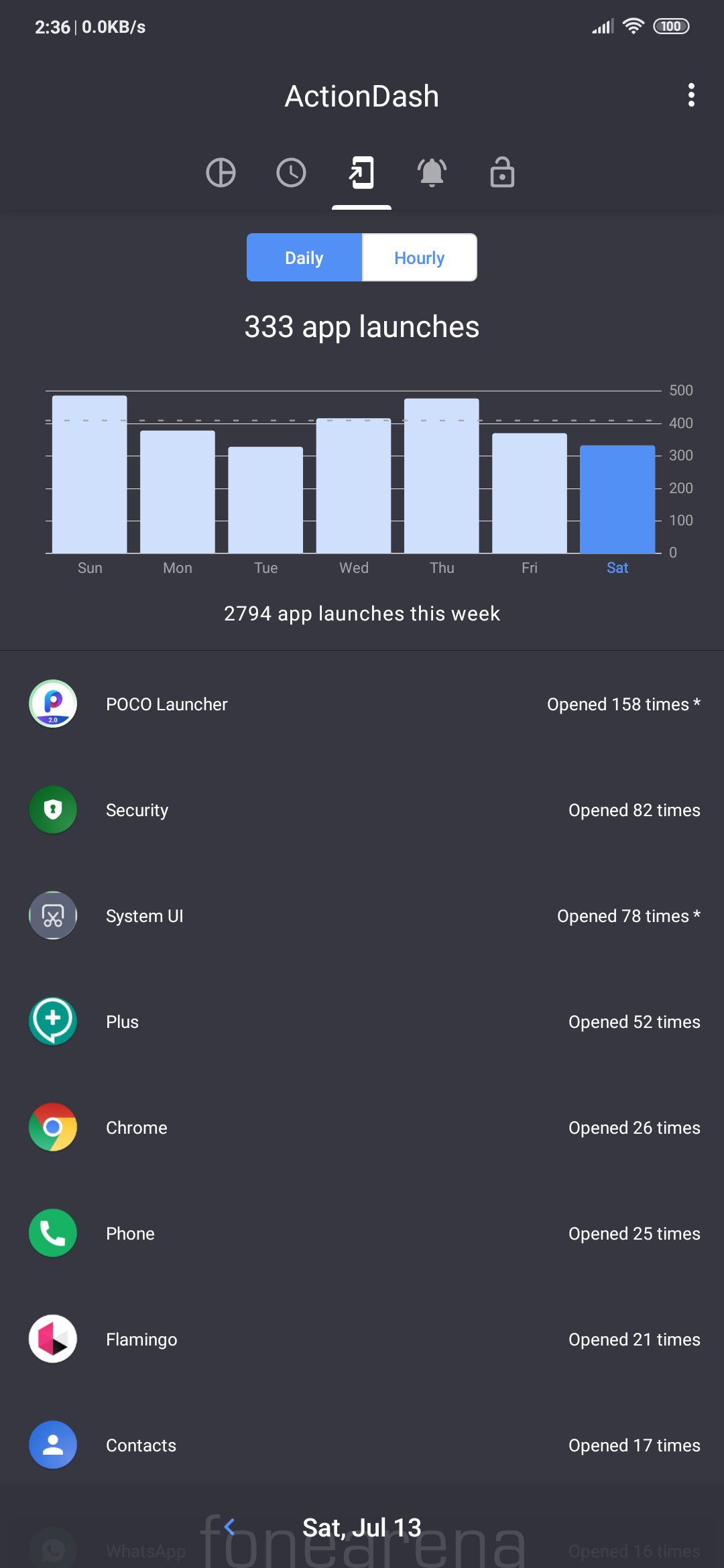A screen capture of a mobile app in portrait mode showcases the Action Dash interface against a dark gray background with white text. At the top, five navigation buttons are displayed, followed by options labeled "Daily" and "Hourly." Under the "Daily" section, it notes that there have been 333 app launches. Below this is a bar graph displaying app launch data for the week, with six light gray bars representing Sunday through Friday and one blue bar on the far right indicating Saturday. The y-axis of the graph ranges from 0 to 500. A total of 2,794 app launches for the week is listed beneath the bar graph.

The lower half of the screen features a detailed list of different apps launched, each with a round thumbnail image to the left and the app name directly to its right. On the far right side is the number of times each app has been opened. The listed apps include Poco Launcher, Security, System UI, Plus, Chrome, Phone, Flamingo, and Contacts. At the bottom of the screen, the date is displayed as Saturday, July 13th.